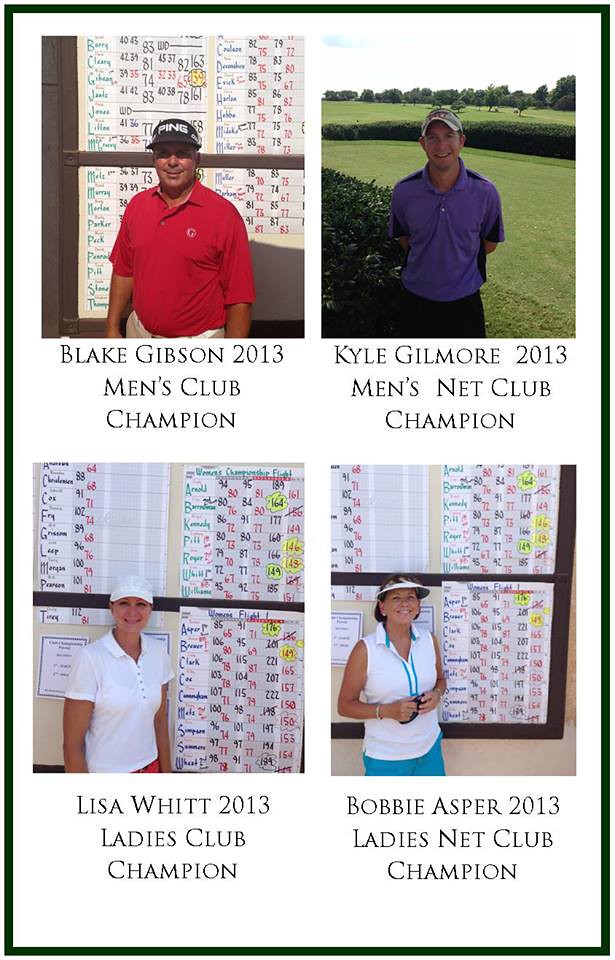The image features four individual portraits, each bordered by a thin black line and arranged in a vertical rectangle, with two men on top and two women below. The top left portrait shows Blake Gibson, identified as the 2013 Men's Club Champion, wearing a black cap with an unclear inscription and a red shirt, accompanied by a background displaying his scores. To the right is Kyle Gilmore, the 2013 Men's Net Club Champion, dressed in a purple shirt and white cap, standing on a golf course beside a bush. The bottom left displays Lisa Witt, the 2013 Ladies Club Champion, in a white cap and shirt, positioned near a chart of her scores. Lastly on the bottom right, Bobby Asper, named 2013 Ladies' Net Club Champion, is seen with a thin black cap exposing the top of her head, a white shirt with blue stripes down the center, and blue pants, holding her arms close to her chest. All four individuals are smiling slightly.